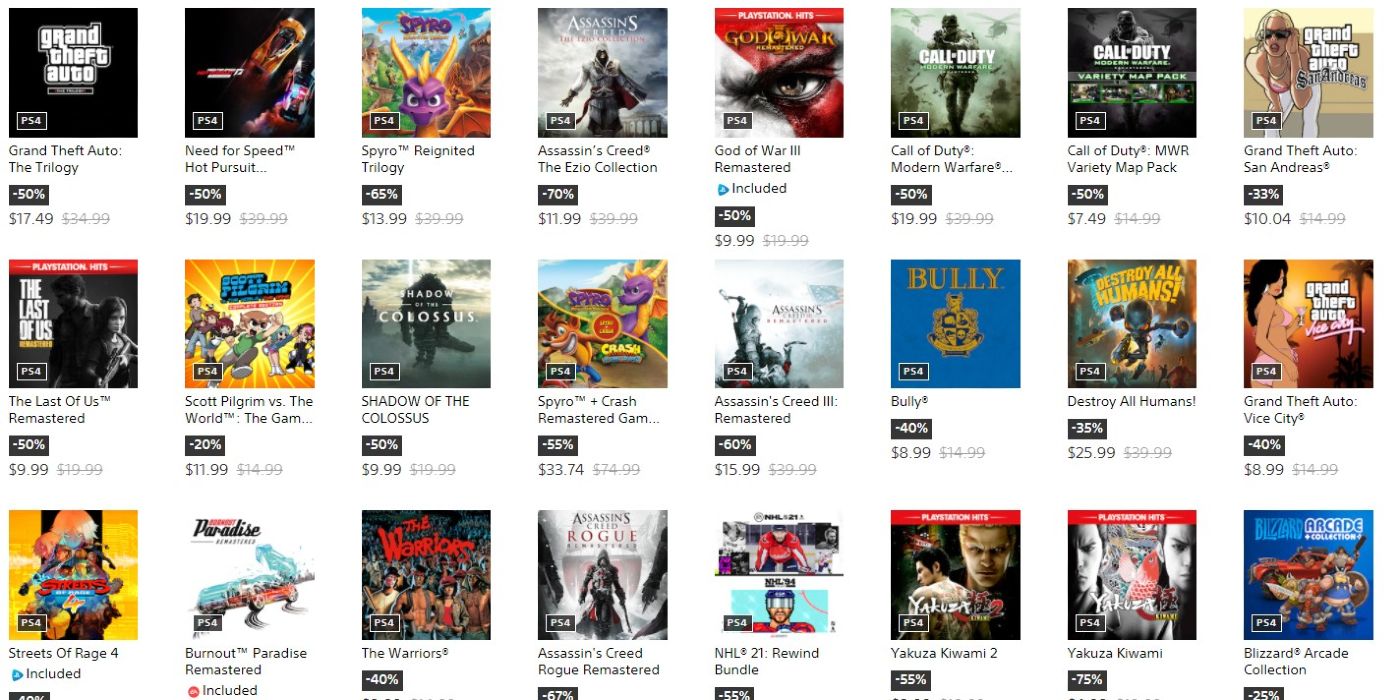A detailed display of a gaming website showcasing video game hard copy sales is presented in three perfectly structured rows. Each row features eight square game cover images, making a total of 24 items listed. From top to bottom, the game titles, discounts, and prices are clearly visible. The first row includes: "Grand Theft Auto: The Trilogy" (50% off, $17.49), "Need for Speed: Hot Pursuit" (50% off, $19.99), "Spyro Reignited Trilogy," "Assassin's Creed: The Ezio Collection," "God of War III Remastered," "Call of Duty: Modern Warfare," "Call of Duty: Variety Map Pack," and "Grand Theft Auto: San Andreas." 

The second row showcases: "The Last of Us," "Scott Pilgrim vs. the World," "Shadow of the Colossus," "Spyro + Crash Remastered," "Assassin's Creed III Remastered," "Bully," "Destroy All Humans," and "Grand Theft Auto: Vice City." 

The final row contains: "Streets of Rage 4," "Burnout Paradise Remastered," "The Warriors," "Assassin's Creed Rogue Remastered," "NHL 21," "Yakuza Kiwami 2," "Yakuza Kiwami 1," and the "Blizzard Arcade Collection." Each game cover is prominently displayed with its title below, alongside the discount percentage and the final price after discount.